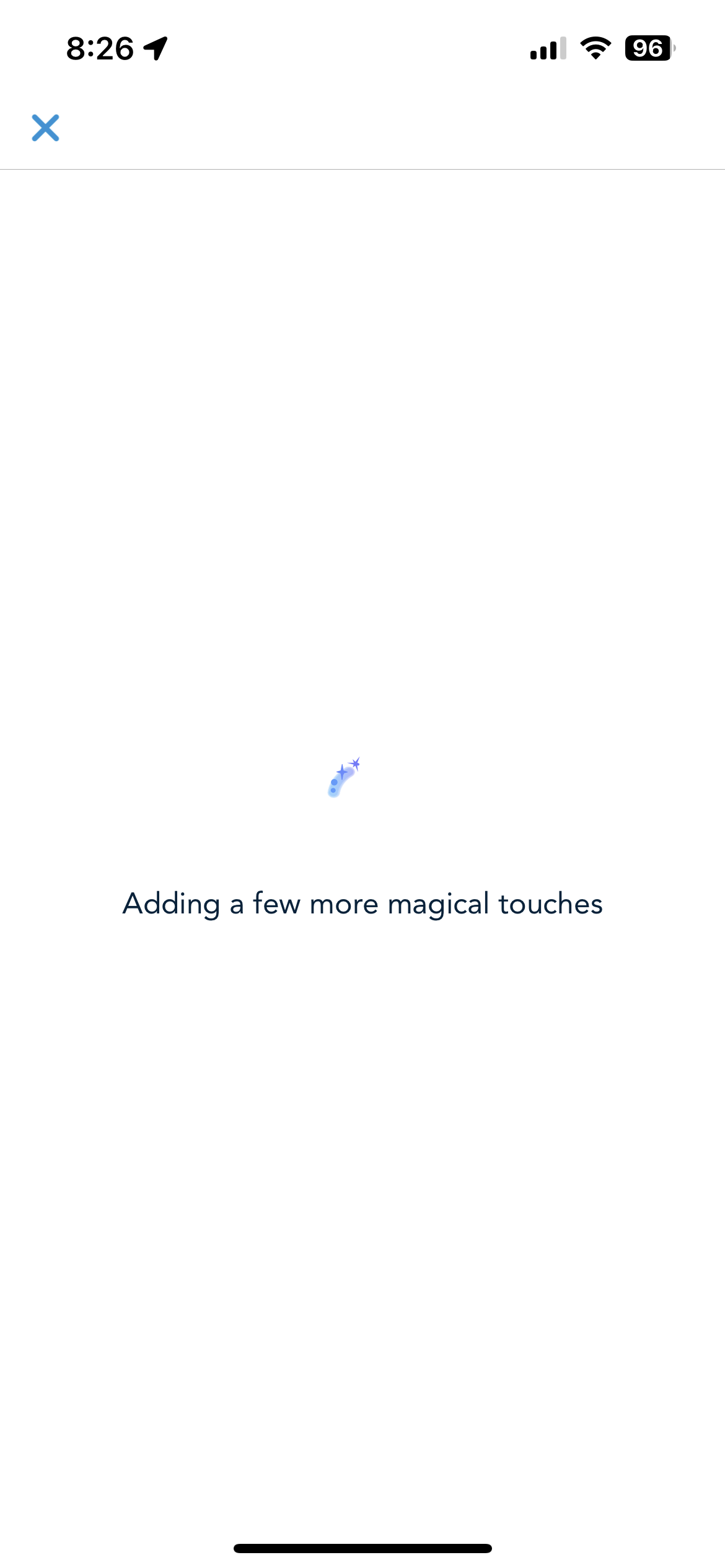This image is a tall and narrow screenshot of a cell phone display. At the top of the screen, the time is displayed as 8:26, accompanied by icons indicating location services, signal strength, Wi-Fi connectivity, and battery life, which is at 96%. A blue "X" icon is located at the top-left corner. The main area of the screen is dominated by a white background. Near the bottom, there is a small glittery swirl, below which the phrase "Adding a few more magical touches" is written. The overall image is simple and lacks photographic or illustrative elements; it contains no people, animals, plants, trees, buildings, vehicles, aircraft, or any other objects. A short black horizontal line is positioned at the very bottom of the screen, concluding the minimalist design.